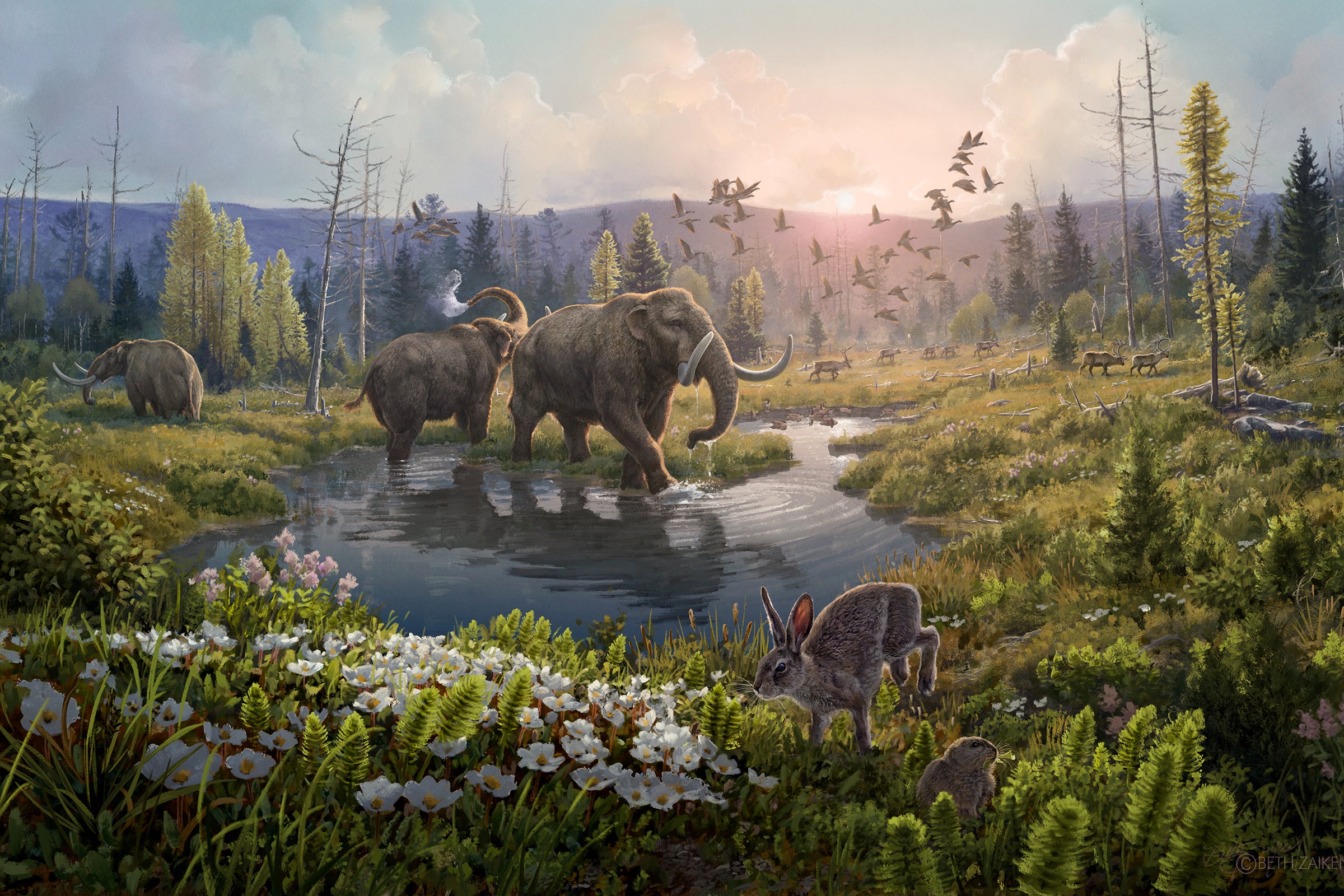This image, resembling a photorealistic painting, captures a serene African landscape teeming with wildlife and lush greenery. At the center is a small pond where three elephants with tusks are milling about; two are wading in the water while a smaller one stands further back to the left. In the foreground, a rabbit moves diagonally to the left among white flowers and greenery. Further back, a flock of birds flies low to the ground. Other indistinct smaller creatures, possibly deer or squirrels, roam in the mid-background. This peaceful scene is set against a backdrop of a distant mountain range, with a cloudy sky occupying the upper fifth of the image, suggesting either dawn or dusk. The detailed flora and fauna create a tranquil and vibrant environment, highlighting the artist's exceptional skill in blending lifelike elements with a painterly touch.